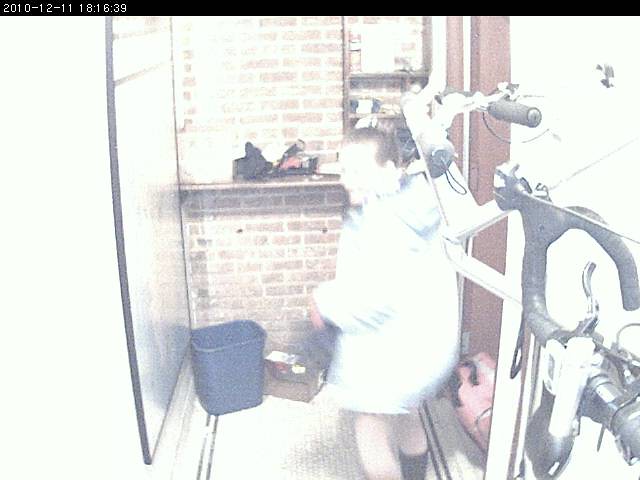In this brightly lit room, a person stands prominently, captured primarily from the left side. He is wearing a white jacket that adds to the well-lit ambiance of the room, paired with black socks that reach up to his calves, and his short brown hair is neatly styled. The room itself is quite detailed with a sliding glass door visible to the left side of the image, beside which a blue trash can is positioned. The backdrop consists of a charming red brick wall, accentuated by a shelf laden with various black items. To the right of the brick wall, brown wooden posts run vertically, along with visible piping and some black pipes interspersed with wires, contributing to a slightly industrial feel.